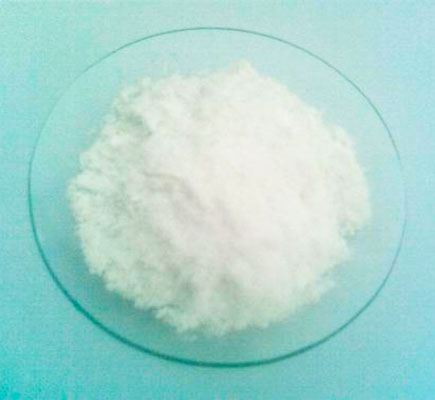This color photograph features a close-up view of a clear glass plate positioned on a turquoise or light greenish-blue tablecloth. Centered on this transparent plate is a sizable, fluffy pile of very fine white powder, resembling the consistency of sugar. The plate's clear nature allows the turquoise hue of the tablecloth to subtly enhance its rim. The background and setting are minimalistic, evoking a laboratory-like environment, and there are no additional objects, people, animals, buildings, or vehicles visible in the image to provide additional context or identification of the powder.